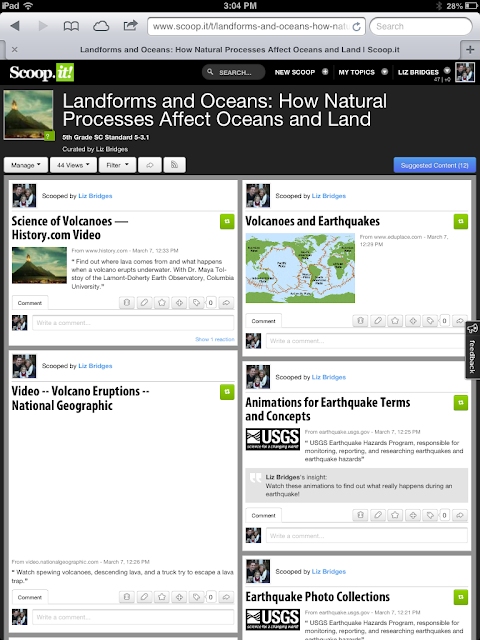An iPad screen displaying Safari is open to a digital curation site called "Scoop.it," focused on educational resources related to geography and oceanography. The iPad's notification area confirms the device type as an iPad. The primary featured article at the top of the page is titled "Landforms and Oceans: How Natural Processes Affect Oceans and Land," labeled specifically for the 5th grade South Carolina standard. Below this main article, the site offers an array of additional resources such as "Science of Volcanoes," a video from History.com named "Volcanoes and Earthquakes" which illustrates tectonic activity, and another video on volcanic eruptions by National Geographic. Many resources are accompanied by the USGS (U.S. Geological Survey) logo, indicating credible scientific backing. Furthermore, the site includes educational animations explaining earthquake terms and concepts, and collections of earthquake photographs. The site appears to be an educational platform aimed at providing children with accessible information on geology and earth sciences.